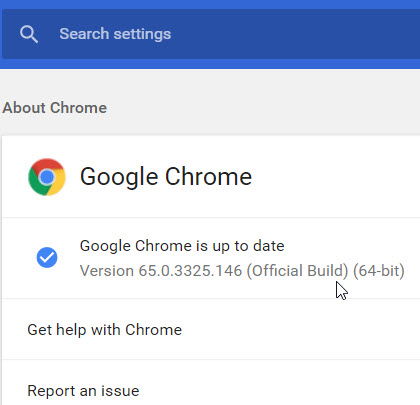A screenshot displays a section of the Google Chrome settings page. At the top, a blue bar contains a magnifying glass icon next to the text "Search settings" in white font. Below this, "About Chrome" is written in gray on a gray background. Prominently featured is the Google Chrome logo, a circle segmented in red, green, and yellow with a blue center. Next to the logo, "Google Chrome" is written in large black font, the most prominent text on the page. Below is a blue check mark followed by the text "Google Chrome is up to date" and the version information, "Version 65.0.3325.146 (Official Build) (64-bit)." Additionally, the page offers a link labeled "Get help with Chrome" and a button for "Report an issue," both set against a white background.